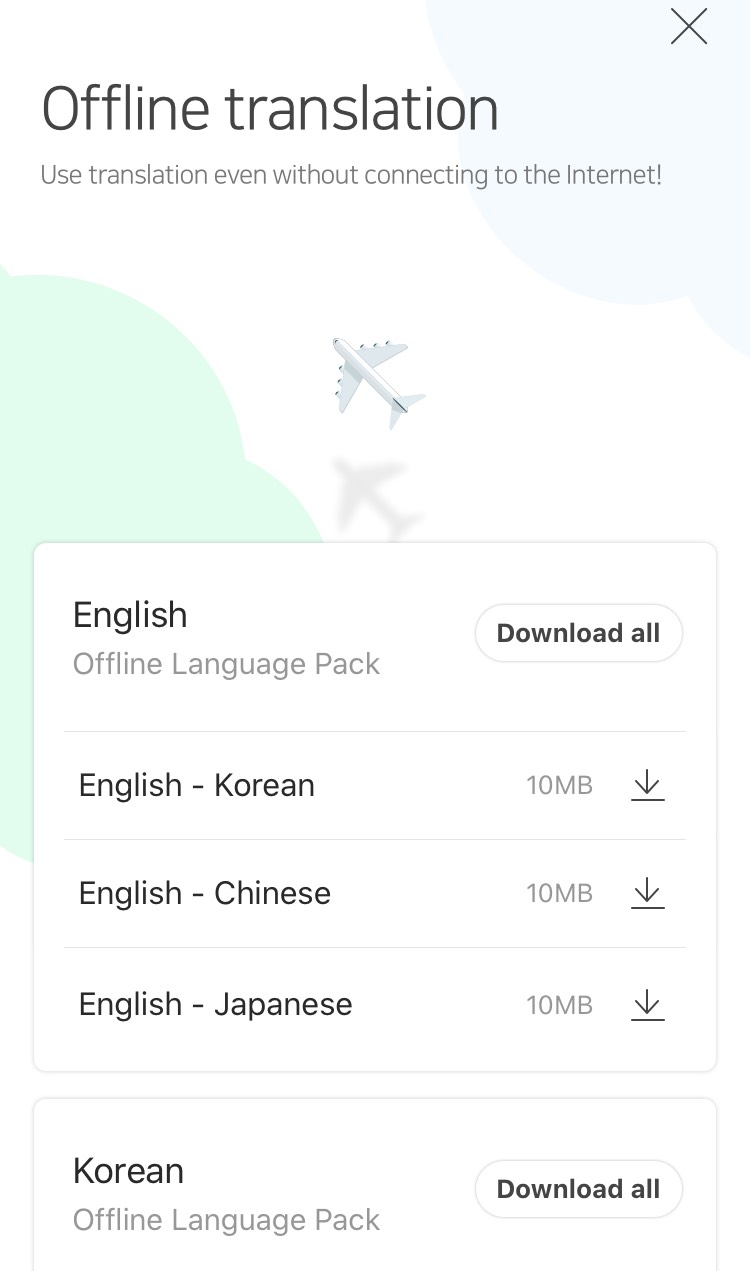This screenshot showcases an offline translation feature, enabling users to access translations without needing an internet connection. The interface is clean and straightforward, characterized by a minimalist design typical of mobile applications.

In the upper right-hand corner, there's a close button. The background image features a plain graphic with subtle shadows and a teal-green cloud-like shape intersecting with two circles on the left.

A prominent white overlay with a border contains the main content. At the top, the word "ENGLISH" appears in bold uppercase letters, followed by "Offline Language Pack" in gray. Below this, several options for download are listed:

- English-Korean: 10 MB (Download button, represented by a downward-facing arrow with a line beneath it)
- English-Chinese: 10 MB (Download button with the same icon)
- English-Japanese: 10 MB (Download button with the same icon)

A "Korean Offline Language Pack" section follows, offering a "Download All" button designed as a white capsule with a thin gray border.

The overall design is streamlined and efficient, with no visible application logos, suggesting it might be part of a phone's system settings or an app developed by a team with good UI/UX knowledge.